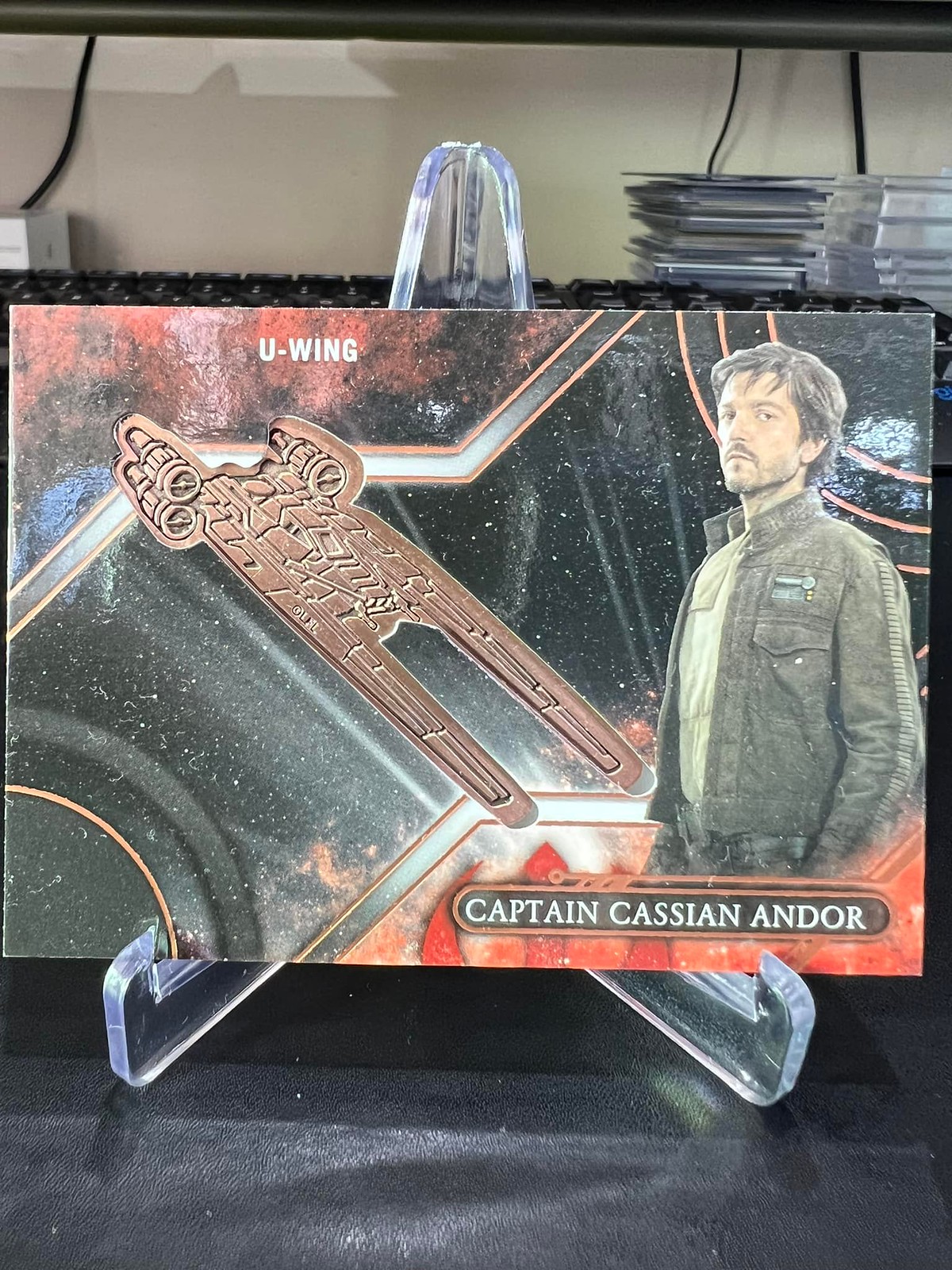This indoor photograph, taken in portrait mode, showcases a detailed and vibrant collector's card from the television series "Andor," part of the Star Wars franchise. The card, mounted on a clear plastic standee atop a black tabletop, features a visual tribute to Captain Cassian Andor, portrayed by actor Diego Luna. Positioned on the right side of the card, Andor, depicted from the waist up, sports a slightly disheveled, straight dark brown hair, a mustache, and a faint five o'clock shadow. He faces left, yet his gaze is directed towards the viewer, wearing a long-sleeve military-style jacket. Below his image, the label "Captain Cassian Andor" is inscribed in white print against a black background outlined in brown.

To the left of Andor's portrait, the card highlights a bronze depiction of the U-Wing spacecraft, distinguished by its four engines and two large U-shaped prongs, resembling a futuristic fork. This design echoes the iconic X and Y wings from the original 1977 Star Wars film. The card's background transitions from red space-themed corners on the upper left and lower right to a black space setting, creating a nebula-like effect across the middle.

Above the collector's card, a shelf can be seen, holding keyboard keys and stacks of trading cards, further emphasizing the image’s detailed and immersive context.